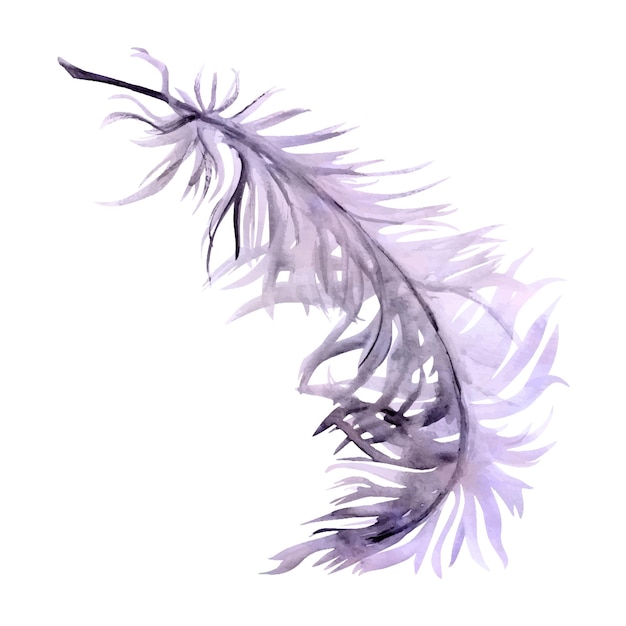This detailed watercolor painting showcases a single, delicate feather with wispy, tendril-like fronds accentuating its frilly structure. The feather, predominantly a lilac purple, subtly transitions through various shades of the color, seamlessly blending and melting into each other. Darker purple streaks and a hint of black in the central quill add depth and contrast. The quill curves gracefully from the top left to the bottom right, with the feather's tendrils seemingly swaying as though caught in a gentle breeze, imparting a sense of movement. Set against a stark white background devoid of any distractions, the feather appears to float, its fronds elegantly dispersed in all directions, enhancing its ethereal and delicate nature.